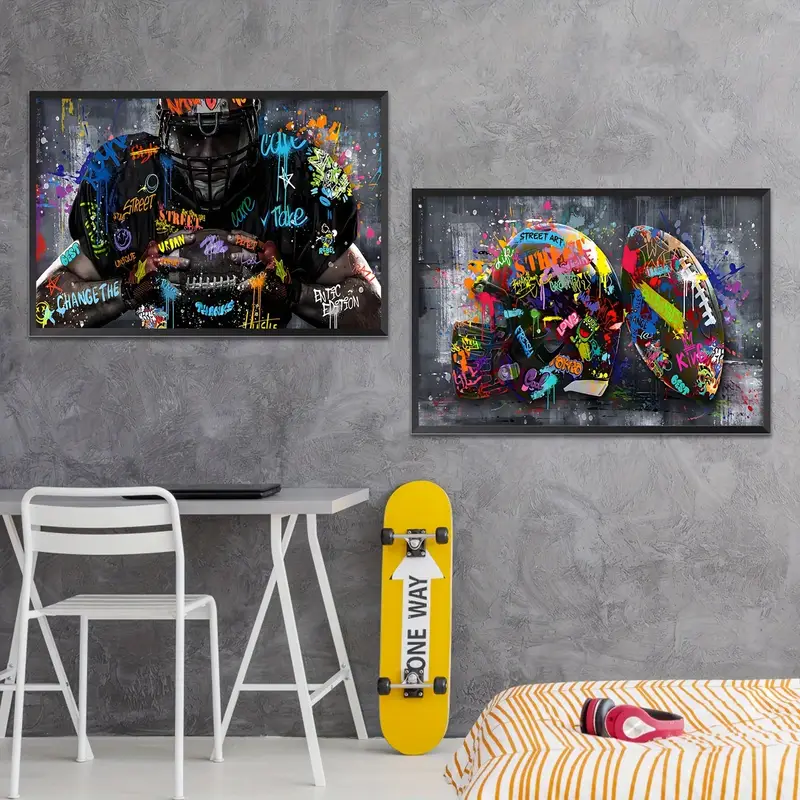The image depicts a modern bedroom characterized by its gray, marble-patterned wall adorned with two framed posters. The left poster features a football player in vibrant Florida Gator colors, covered with a collage of abstract paint splashes and words like "change the" and "street urban intake," rendered in shades of turquoise, orange, yellow, blue, and green. The right poster mirrors the style of the first, showcasing a football helmet and football, with similarly colorful and abstract elements. Positioned below these posters is a sleek white desk accompanied by a white metal chair and a black laptop. To the right of the desk stands a yellow skateboard, propped vertically against the wall, with the words "One Way" in dark gray letters and an arrow pointing up. To the right of the skateboard is a bed topped with a white comforter featuring bold orange stripes. Resting atop the comforter are a pair of red wireless headphones with gray accents. The room is captured in a style reminiscent of a stock photo, aiming to showcase its clean, modern aesthetic.